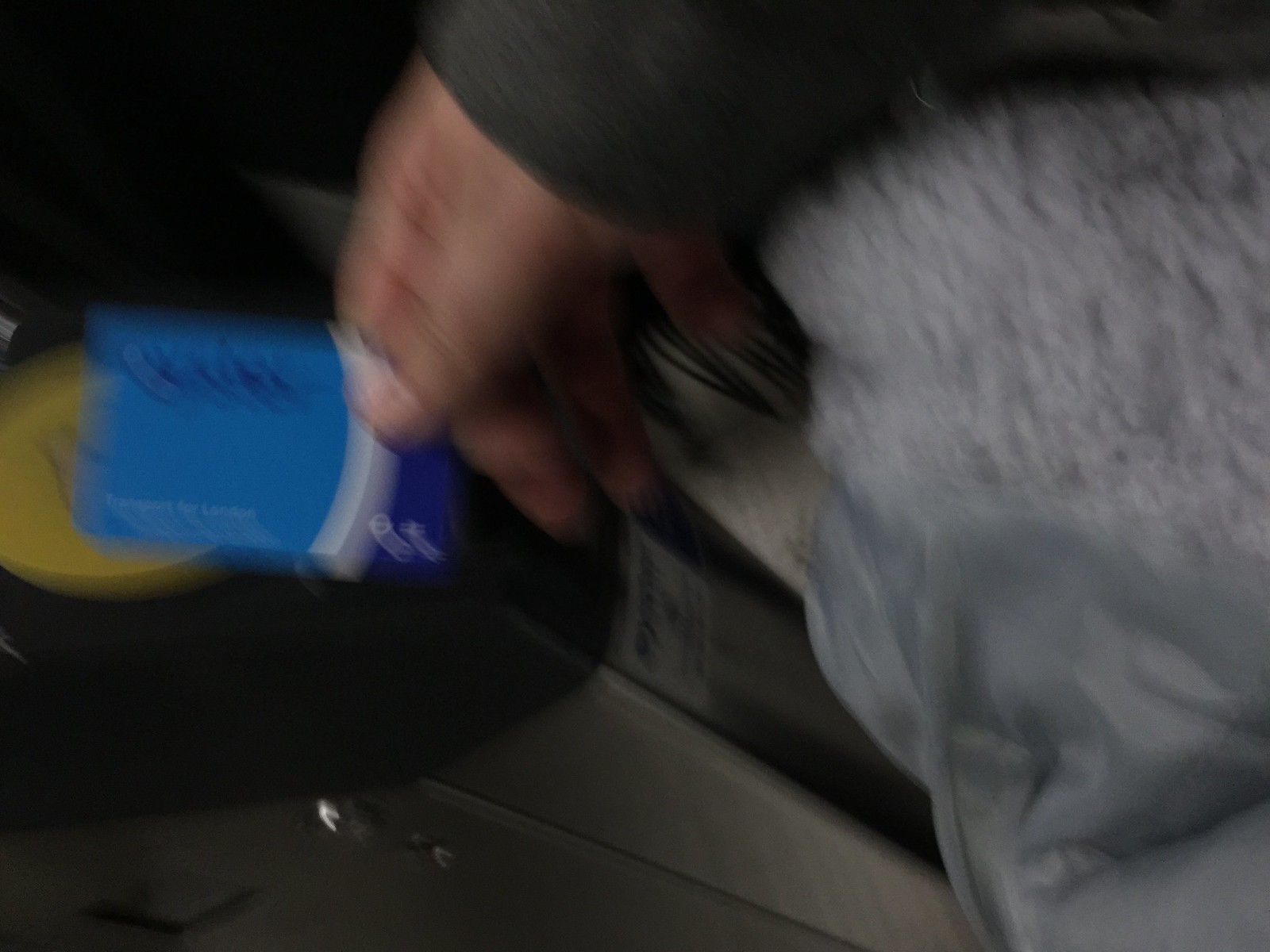A blurry photo captures a person's hand about to tap a light blue plastic card onto a yellow circle, possibly for contactless payment. The card features a white stripe transitioning to a dark blue edge on the right. The individual’s hand, with fair skin, emerges from the sleeve of a black coat. The scene’s background includes a white-grayish carpet or upholstery to the right side of the frame, adding to the overall context.